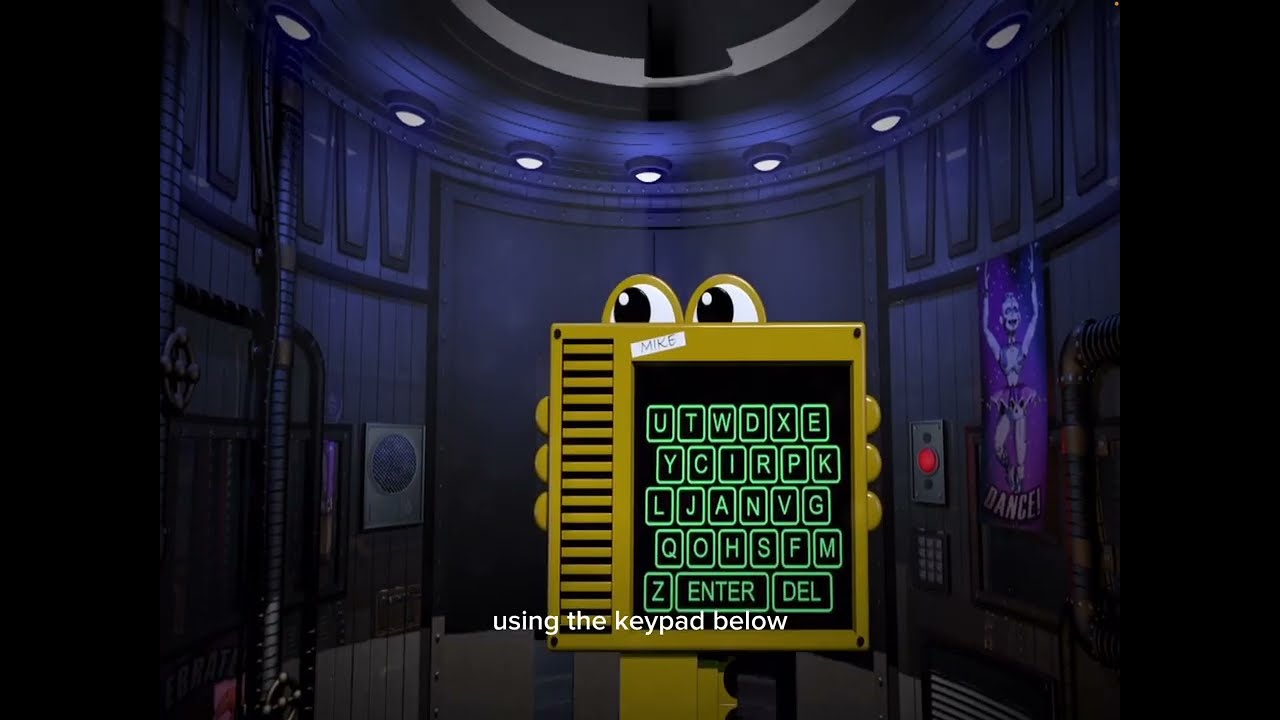The image is a detailed, vibrant scene from a cartoonish video game setting, depicting a rounded chamber, perhaps resembling a spaceship's interior. The central focus is a mustard-yellow keypad device with a speaker on the left side and two cartoonish eyes at the top, reminiscent of alligator eyes peeking over. The keypad, located centrally, displays a dark screen with green lettering that spells out: "U-T-W-D-X-E," "Y-C-I-R-P-K," "L-J-A-N-V-G," "Q-O-H-S-F-M," and "Z," along with clearly marked "enter" and "delete" buttons. 

Above the screen, white text states, "use the keypad below." The background is primarily dark black with what appear to be metal walls, featuring brown and white sections towards the floor and recessed lights forming a circular pattern on the ceiling. 

On the right-hand side of the chamber is a purple poster of a cartoon robot in a tutu, bearing the word "Dance" in white text. Adjacent to the poster, slightly to the left, is a silver panel with a red button. The setting’s design elements, along with the specific colors of black, white, gray, purple, red, yellow, and green, contribute to the overall whimsical and engaging atmosphere of the scene.